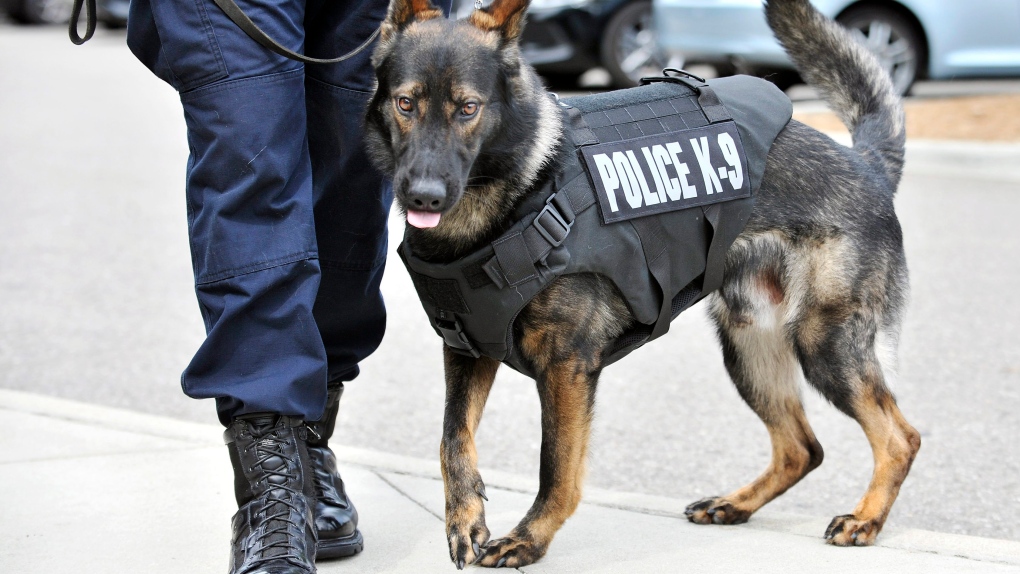This detailed photograph features a vigilant police canine and its handler depicted in a street setting. The canine, a dark-colored German Shepherd, is adorned in a black nylon vest emblazoned with "POLICE CANINE" in white letters. The dog's snout is black, and its eyes are a striking yellowish-brown. Its tongue peeks out slightly as it gazes directly at the camera, exuding readiness and alertness. Positioned on its left, the handler is partly visible from the boots up to the mid-thigh, donning dark blue military-style pants and black combat boots laced up the front. The handler is holding a black leather leash that attaches to the dog's vest. The duo stands on a concrete surface with a light blue car and a dark blue car visible in the background, suggesting they are on a sidewalk adjacent to a road. The dog's posture and expression indicate it is poised and prepared for action.